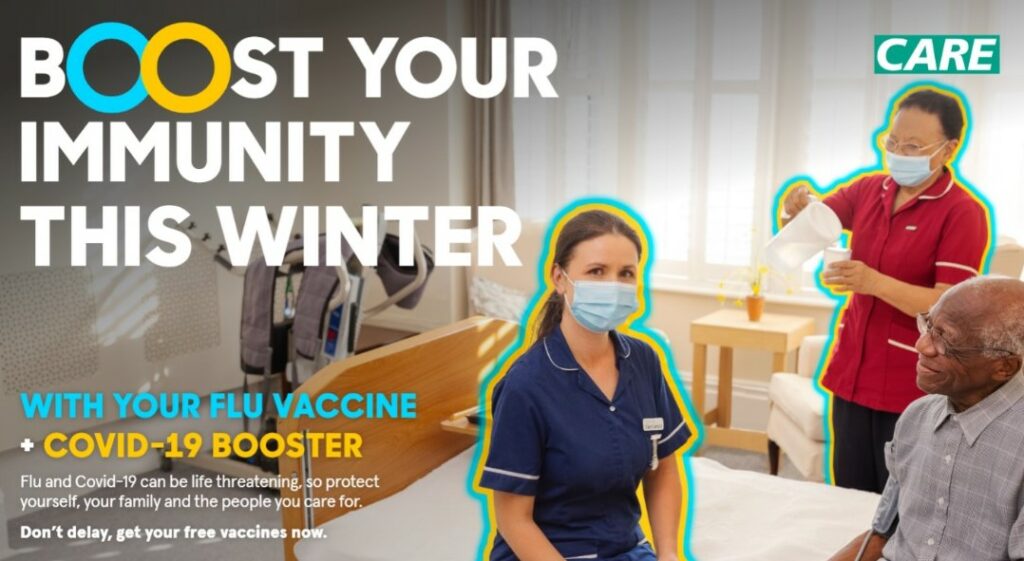This is a web advertisement for healthcare focusing on immunity protection this winter. The top left-hand corner features text that reads "Boost your immunity this winter," with the O's in "boost" enlarged, one in blue and the other in yellow. Underneath, the text says "with your flu vaccine and COVID-19 booster," with "flu vaccine" in blue letters and "COVID-19 booster" in yellow. Below that, it reads, "Flu and COVID-19 can be life-threatening, so protect yourself, your family, and the people you care for. Don't delay, get your vaccine now."

The ad's photograph is set in a well-furnished room resembling a hospital or nursing home. In the foreground, a nurse dressed in blue scrubs, with her brown hair pulled back in a ponytail and wearing a blue face mask, sits on a bed. An elderly African-American man with glasses, a bald head, and a gray checked button-down shirt, featuring a blood pressure cuff on his right arm, sits beside her, smiling at her.

In the background, another nurse in red scrubs with a blue mask is seen pouring water into a cup. Behind her are an easy chair, a wooden table, and large windows, adding a comfortable ambiance to the setting. Partially obscured by the text, there appears to be medical equipment, possibly a treadmill or walker, on the left side of the room. This detailed setting aims to convey a comprehensive message about the importance of getting vaccinated for flu and COVID-19 to stay protected during the winter season.